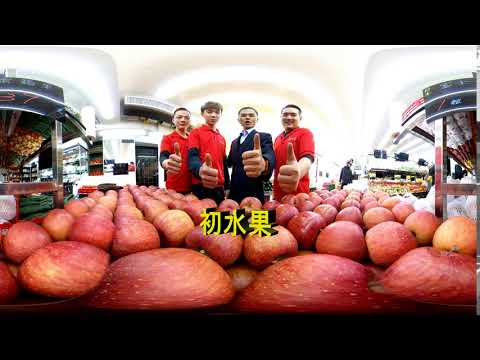In this vibrant, fisheye-lens image, four individuals, three in red polo shirts and one in a navy suit jacket and white collared shirt, are standing inside a brightly lit grocery store. Each person is giving a cheerful thumbs up to the camera. The store is bustling, with various produce stands and shoppers visible in the background, emphasizing the lively atmosphere. The foreground prominently features a table brimming with red and orange apples. Notably, yellow Asian characters are situated in the center of the frame, adding a touch of cultural texture to the scene. Within this diverse setting, white walls and metal shelves further define the supermarket’s interior, suggesting a well-organized and clean environment.